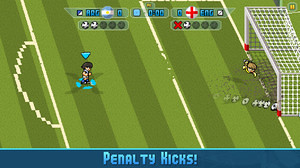In this image depicting a classic video game, we observe a small, rectangular screen. At the bottom, there is a thick blue bar with a lighter blue line above it. In the middle of this bar, the words "PENALTY KICKS" are displayed in all caps, with the "P" and "K" slightly larger than the other letters.

The central part of the screen shows a digital soccer field, marked by alternating light and olive green lines that are just over a centimeter wide. Positioned on the right-hand side is a white goal net, with a soccer ball visible in front of it, suggesting that it is about to enter the net.

In the foreground, a partially visible player — seen only from the head and part of the arm due to the angle — appears to be in a defensive position near the net. On the left-hand side, another player, who seemingly took the shot, is surrounded by small blue lights around his feet.

At the top of the screen, numerical indicators and small soccer ball icons display the current score, encapsulating a decisive moment in this digital soccer match.